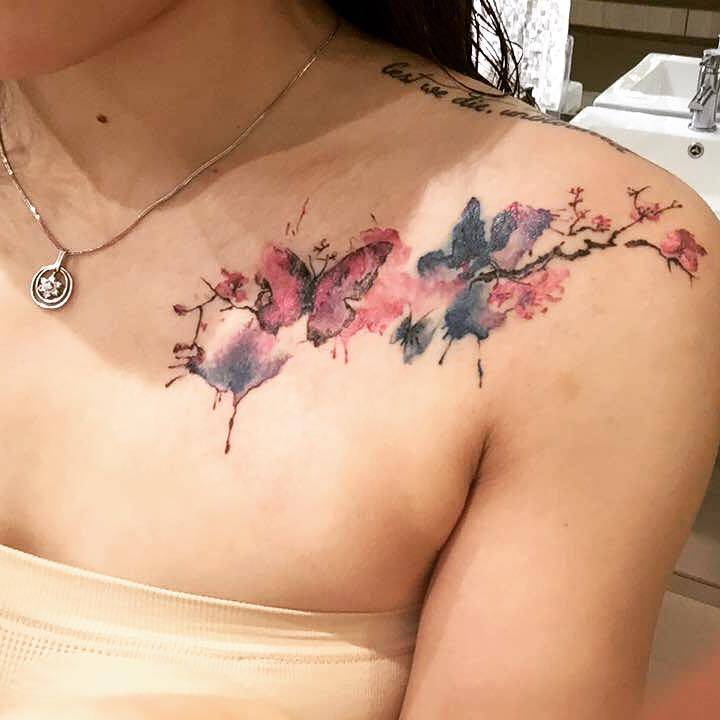In the image, we see a young Caucasian woman, predominantly showing her left shoulder, neck, part of her chin, and her upper chest region. She is wearing an off-white, beige-colored shirt. Adorning her neck is a silver necklace, which features a circular pendant with an intricate design that appears to be either a star or a flower, possibly resembling a snowflake. 

The focal point of the image is her tattoo, which starts on her chest and extends across her shoulder blade. This intricate tattoo includes splotches of red coloration, resembling blood splatters, which transition into vine-like branches adorned with buds, and includes two butterflies. One butterfly is a pinkish-red in color, while the other has a darker, navy blue hue. The overall aesthetic of the tattoo gives a watercolor painting feel.

Additionally, she has another tattoo at the very top of her shoulder bearing some barely legible script, possibly in French, with what might be the phrase "C'est Di...". Behind her, there is a white sink with a silver faucet, and a mirror reflecting her image, indicating that she might still be in the tattoo parlor where she got her tattoo.